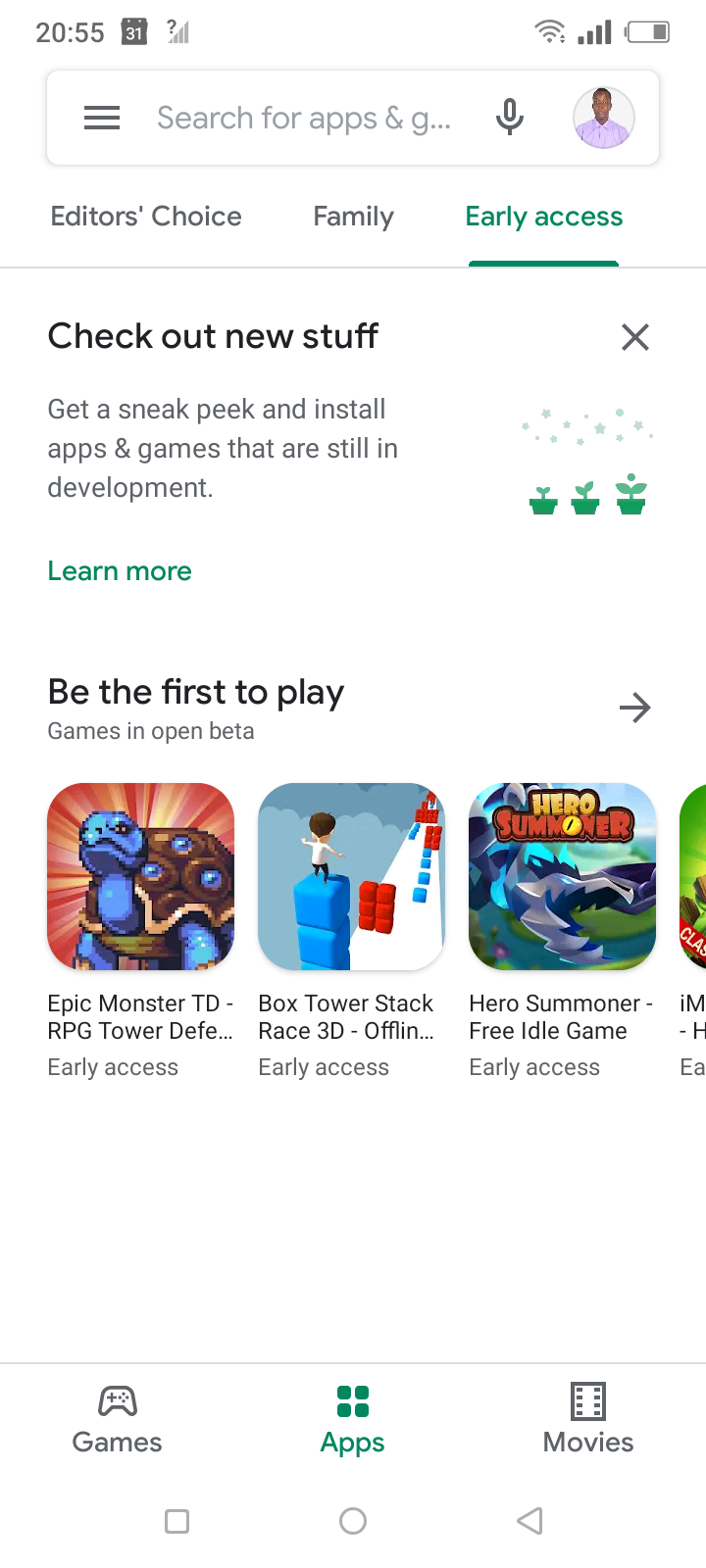"Screenshot of a smartphone display captured at 20:55 on the 31st of the month. The phone has full four bars of signal strength and Wi-Fi connection, with the battery level at approximately 25%. At the top of the screen, a hamburger menu icon and a 'Search for apps & games' bar with a 'G..' partially visible, followed by a microphone icon and a human avatar icon are displayed. Below these, there are three horizontally aligned menu options: 'Editor's Choice,' 'Family,' and 'Early Access,' with 'Early Access' highlighted in green and underlined, while the other two are in gray.

Underneath the menu options, a gray notification banner appears with the message 'Check out new stuff' adjacent to a close button (X) on the right. Below that, the text explains, 'Get a sneak peek and install apps and games that are still in development,' accompanied by a graphic of growing plants. The words 'Learn more' are highlighted in green below this explanation. Further down, it states 'Be the first to play games in open beta,' followed by a right arrow icon.

Four app icons are listed below this section: 
1. 'Epic Monster TD, RPG Tower Defense' marked with 'Early Access.'
2. 'Box Tower Stack Race 3D.'

The rest of the app names are truncated and appear as 'DEFE...' and so on."